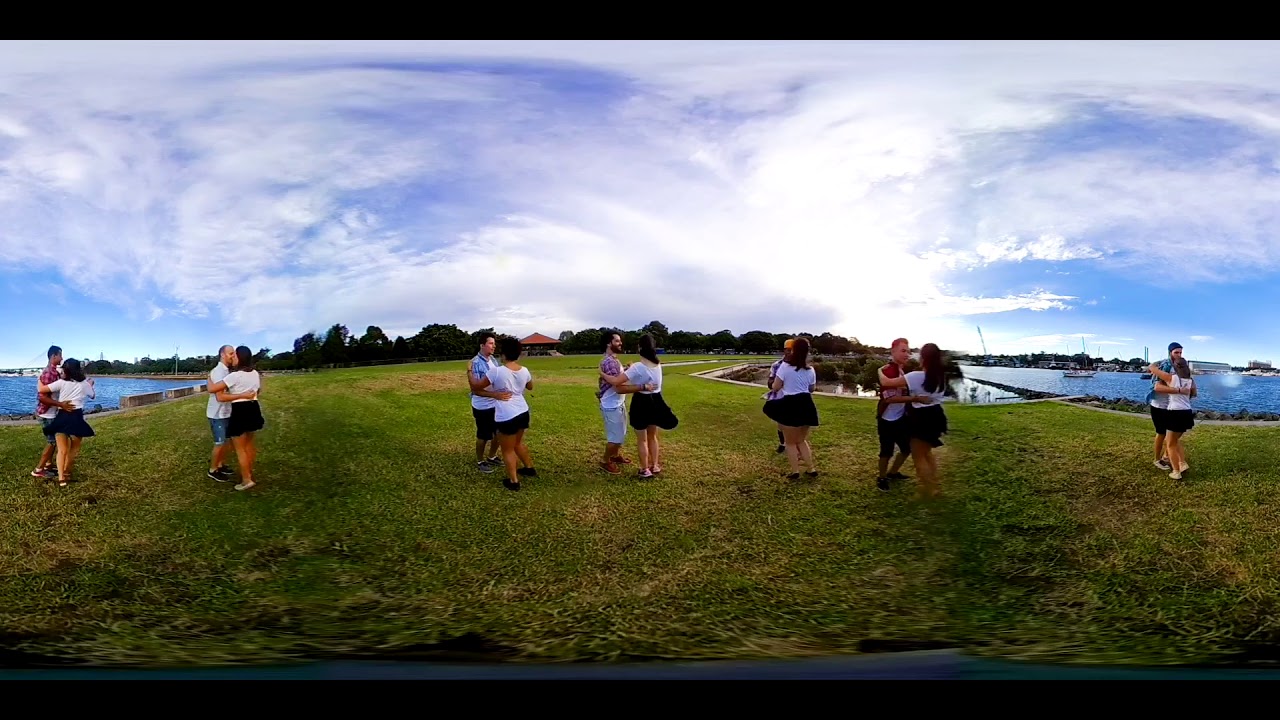In this vibrant color photograph, seven couples are gracefully dancing on a grassy field that stretches between two bodies of deep blue water. Each woman is dressed in a white shirt and black shorts, paired with men who sport shorts and a variety of colored shirts in shades of red, white, and blue. The couples are arranged in a line, dancing together in the center of the image. To the left and right of the grassy strip, you can glimpse the water, dotted with white sailboats on the right.

In the background, a picturesque scene unfolds with lush, green trees surrounding a small building with an orangish-brown, pointy roof, which resembles a gazebo or shelter. The sky above is a serene blend of light blue and swirling white clouds, creating a partly cloudy atmosphere. This captivating image, possibly of a dance class held in a park-like setting, captures the harmonious interaction of natural elements and human activity.